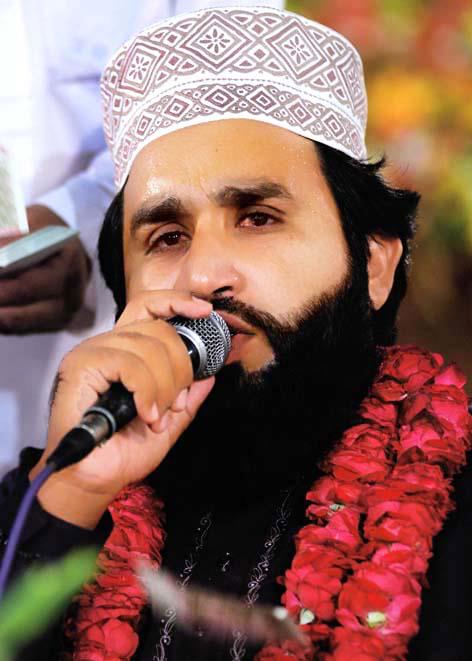This vertically oriented photograph prominently features a man, visible from the chest up, who appears to be a religious figure possibly delivering a speech. He is wearing a patterned cylindrical hat adorned with diamond shapes that contain flowers, set against a background of gray, purple, and white. His light brown skin is framed by a thick black beard and mustache, with black hair emerging from under his hat. The man dons a black outfit accentuated by two vibrant red floral garlands around his neck. In his left hand, he holds a microphone with a silver top, black handle, and purple wire, which he is speaking into. In the background, to the left, stands another man with dark brown skin, wearing a white shirt and holding a piece of paper, his face not visible. The backdrop features a mix of green, red, and yellow hues. The image captures the essence of a religious or public speech given by a distinguished figure.